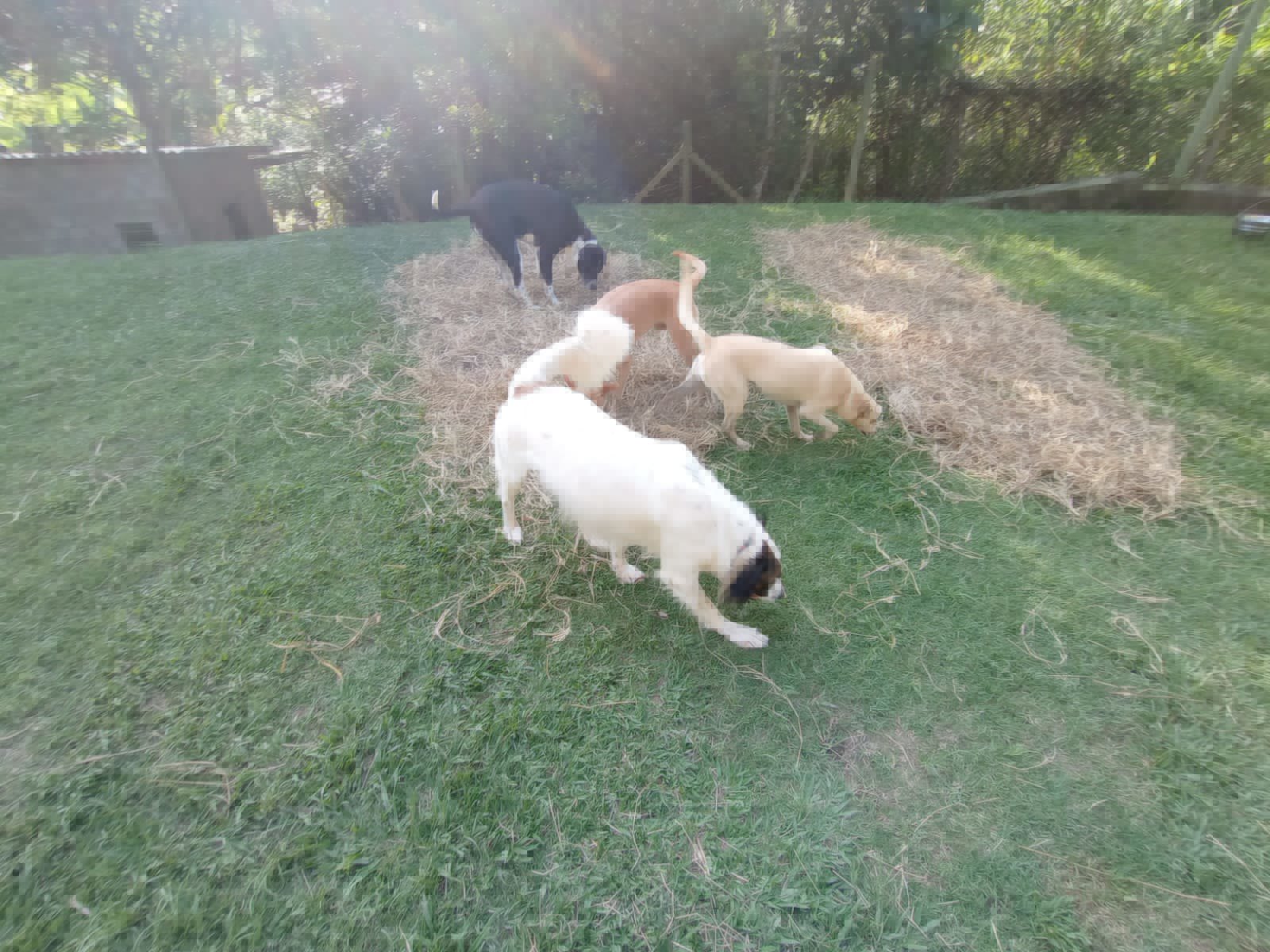In this slightly blurry, low-resolution photograph, taken in a horizontal orientation, the setting is an outdoor yard featuring a scene filled with lush greenery and dappled sunlight. The foreground is dominated by a lawn covered in freshly cut grass with patches of dry clippings. At the center, two tan-colored stripes of hay stretch approximately 6 feet wide by 12 feet long, bordered by strips of green grass. The scene is lively, with four medium-to-large dogs, each engrossed in sniffing the ground. The dogs include a white one with a distinct black and tan face, a tan one, a brown one, and a black one with white markings on its chest, paws, and neck. A fifth dog is in the background. 

The background, occupying the top quarter of the image, is a verdant landscape of trees and shrubs. To the left side of the photograph, a small light brown shed or building is partially visible. Additional elements in the backdrop include a mix of wooden and brick fence segments, some power poles, and scattered wooden poles. The slightly hilly terrain appears to slope gently downward toward this eclectic scene's left side, enhancing the rustic charm of this backyard tableau.